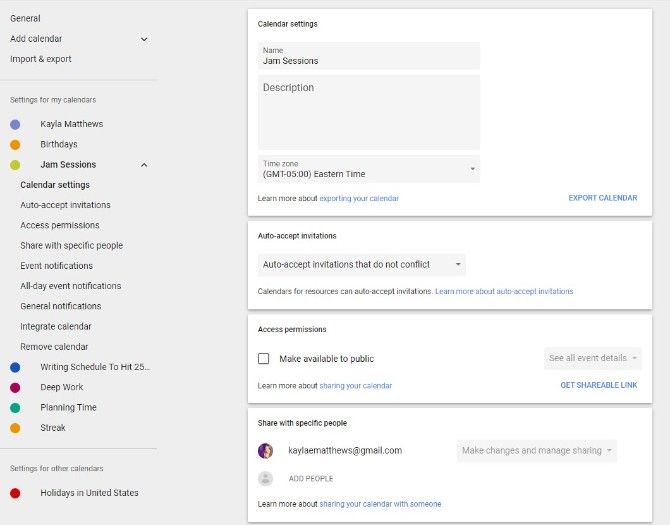This image is a screenshot of a website featuring a detailed view of calendar settings. The background of the page is light gray. On the left side of the screen, there is a menu with various options listed. At the top of the menu, highlighted in dark text, is the word "General". Below that, you find "Add Calendar" with a drop-down menu, followed by "Import and Export". Further down, the menu reads "Settings for My Calendars", including specific listings such as "Kayla Matthews", "Birthdays", "Dream Sessions", "Calendar Settings", "Auto Accept Invitations", "Access Permissions", "Share with Specific People", "Event Notifications", "All-Day Event Notifications", "General Notifications", "Integrate Calendar", "Remove Calendar", and entries labeled "Writing Schedule to Hit 25", "Deep Work", "Planning Time", and "Streak". 

Additionally, under "Settings for Other Calendars", there is "Holidays in the United States".

On the main part of the screen, which has a white background, the heading "Calendar Settings" is displayed in black text at the top. Below this heading is a gray banner that labels the section "Name" with the following text "GM Sessions". Following some space, there appears another gray banner labeled "Background". Under this, the term "Descriptions" is displayed. Below that, it notes the "Time Zone" as "GMT-05:00" with "Eastern Time" in parentheses, followed by a drop-down menu. 

Further information on the page includes a section labeled "Learn more about exporting your calendar". Under the "Auto Accept Invitations" subsection, it specifies "Auto Accept Invitations that do not conflict" with a drop-down menu. 

The "Access Permissions" section includes options such as "Make Available to Public" and another link titled "Learn more about sharing your calendar". Within this subsection, it states "See All Event Details" and "Get Shareable Link". 

Continuing down, under the "Share with Specific People" section, an email address is listed: "Kayla E. Matthews at gmail.com", with additional options to "Add People", "Make Changes, and Manage Sharing", accompanied by a drop-down menu.